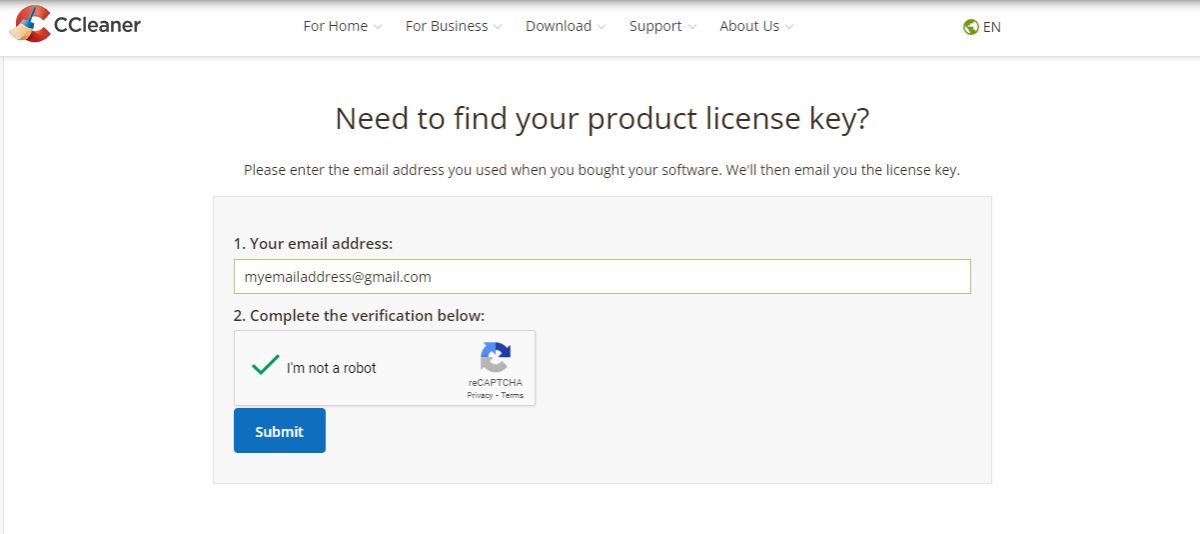This image depicts the user interface of the CCleaner website. In the upper left corner is the CCleaner logo, featuring a prominent, red letter 'C' wrapped around the handle and bristles of a broom. To the right of the logo, the brand name "CCleaner" is displayed in black text.

Stretching across the top of the interface, there's a navigation bar offering multiple links, including "Home," "For Business," "Download," "Support," and "About Us." On the far right of this bar, there is an option marked with "EN" next to a globe icon, representing language options with English selected.

The main section of the page is dedicated to helping users retrieve their product license key. It prompts users to enter the email address they used during the purchase. There is a light gray rectangular input field labeled "1. Your email address," where users are supposed to type their email. An example email like "myemailaddress@gmail.com" is provided for clarity.

Additionally, the section requires completion of a CAPTCHA for verification, labeled "2. Complete the verification below." This involves an interaction step where users click on images to prove they are not a robot.

Beneath these input fields is a prominent blue rectangle button with white text that reads "Submit," allowing users to submit their email address to receive their license key.